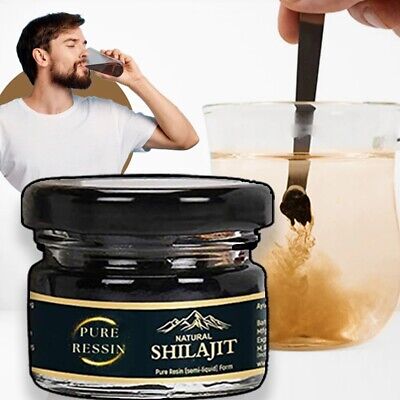This advertisement for Pure Resin Natural Shilajit Pure Resin showcases a small, round, black glass jar prominently labeled with the product's name, positioned at the forefront. To the right, a see-through glass cup filled with water is being stirred by a black stirrer held by a Caucasian hand, visibly dissolving the resin and turning the water slightly brown. On the left, a man with dark hair and a beard, dressed in a white t-shirt, is depicted drinking a cup of the brown liquid. The cohesive setup emphasizes the transition from the black jar of resin to its mixed liquid form, highlighting the product's use and appeal.